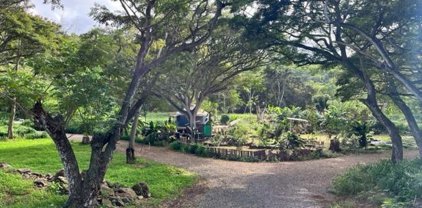This color photograph, captured in landscape orientation, depicts a serene park scene during the daytime. The focal point is a dirt walking path with a light brown pebble finish that branches off to the left and right, creating a natural fork. This path is enveloped in greenery with tall trees on both sides, growing towards the middle to form a leafy canopy, providing ample shade. In the center of the image, there is a garden area with shrubs and flowers, adding to the park's tranquil atmosphere. The left side of the path is characterized by a large tree with low branches and smaller trees, presenting a more child-friendly, grassy section. In contrast, the right side appears more sparse, leading into an open field. The photograph, taken either in the early morning or under a cloudy sky, offers a realistic and panoramic view of this lush, arboretum-like setting.